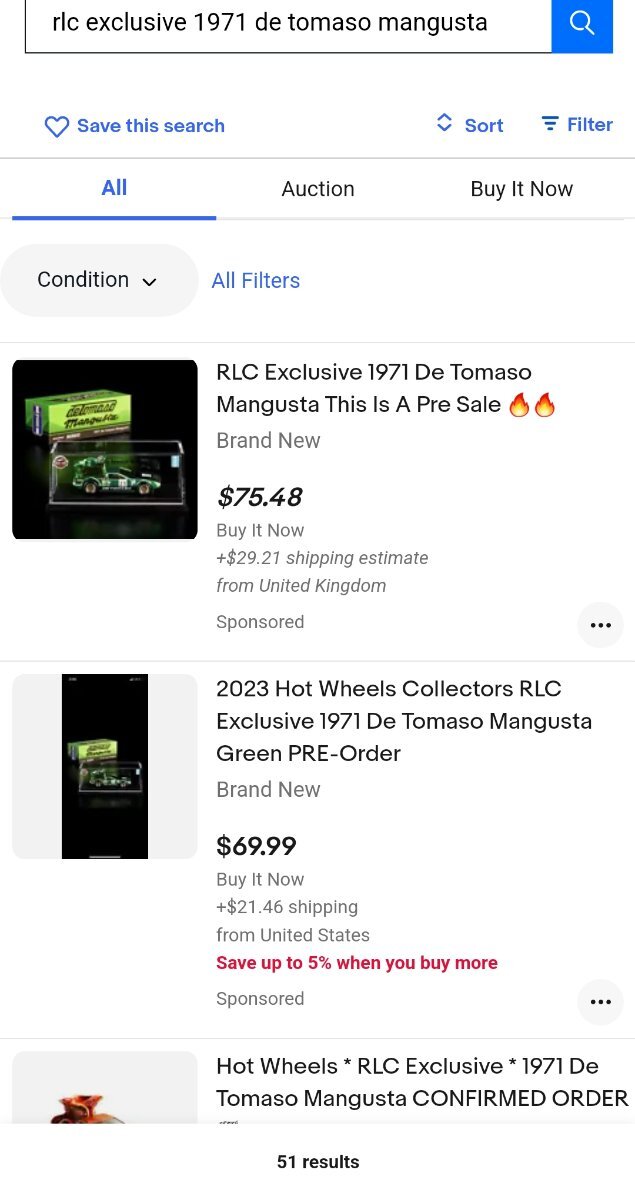This is a detailed caption for the provided image description:

---

The screenshot displays a website interface dedicated to selling various items. At the very top, there is a white search bar outlined in black, accompanied by a blue search button, prominently indicating "RLC Exclusive 1971 D. Tommaso Mangusta." Below the search bar, in blue text, options for "Save this search," "Sort," and "Filter" are visible. Beneath these options, a navigational line allows users to toggle between "All," "Auction," and "Buy It Now," with "All" currently selected and highlighted in blue.

Directly under this navigation line, there is an additional filtering option labeled "Condition," followed by an "All Filters" button, both displayed in blue. The main content area reveals three item listings, though only two are fully visible. 

The first listing features a black box showcasing a detailed image of the "RLC Exclusive 1971 D. Tommaso Mangusta" model car. This listing is marked as a pre-sale and is adorned with two small fire icons, indicating high interest or limited availability. The price is listed as $75.48, with a "Buy It Now" option. The estimated shipping cost is an additional $29.21 from the United Kingdom. The listing is also tagged as "Sponsored."

The second listing appears to offer a similar item but with slight variances in the presentation. It showcases the "2023 Hot Wheels Collectors RLC Exclusive 1971 D. Tommaso Mangusta" in green. This item is also described as a pre-order and brand new. The price is listed at $69.99 with "Buy It Now" and an estimated shipping cost of $21.46 from the United States. Additionally, there is an offer to save up to 5% on multiple purchases, and this listing is also marked as "Sponsored."

Further listings, including another Hot Wheels item, are partially visible but not fully described.

---
This caption thoroughly integrates the elements and details from the original image to provide a comprehensive and clear description.